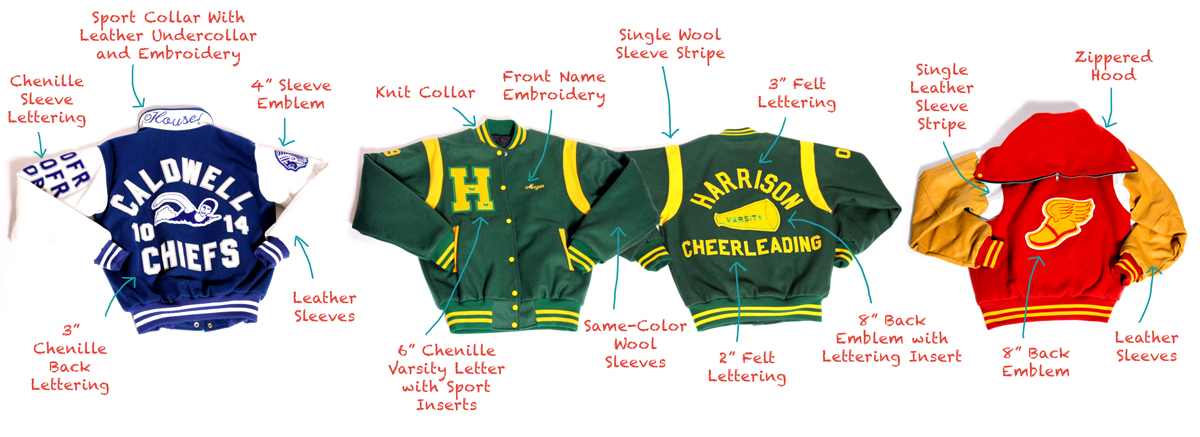The image showcases four distinct sports jackets against a predominantly white background, with detailed annotations pointing to various features in red text and blue arrows. From left to right:

1. A blue and white jacket labeled "Caldwell Chiefs" featuring a sport collar with leather under-collar, chenille sleeve lettering, chenille back lettering, leather sleeves, and a four-inch sleeve emblem in red.

2. A green jacket with a letter "H" and yellow stripes identified as "Harrison Cheerleading" with a knit collar, front name embroidery, single wool sleeve stripe, same color wool sleeves, two and three-inch felt lettering, and an eight-inch back emblem with lettering insert.

3. Another green variant similar to the Harrison jacket but with distinguishing features like six-inch chenille varsity letters with sports inserts.

4. A red and orange jacket with leather sleeves, single leather sleeve stripe, zippered hood, and an eight-inch back emblem featuring a winged foot.

Overall, the photo highlights varsity jackets for kids, emphasizing the mix of colors and detailed customization options.